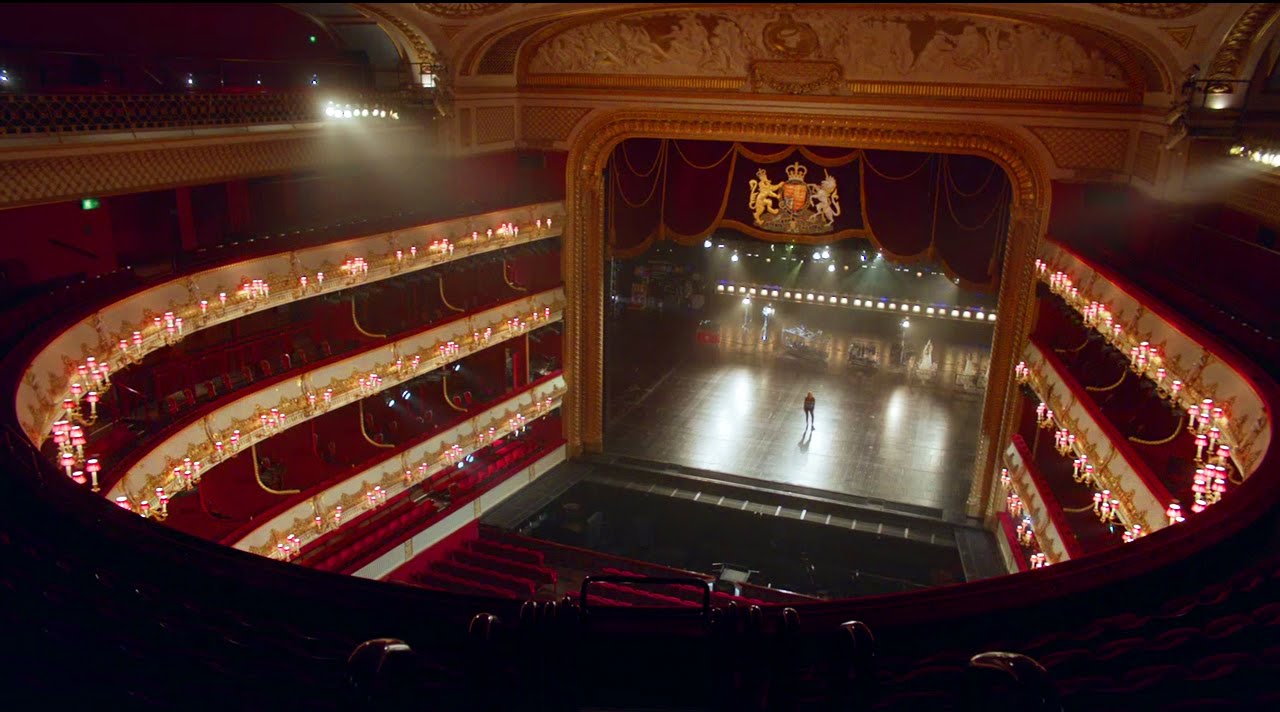The image depicts an elaborate and grand auditorium viewed from an upper level, looking downward towards the stage. The auditorium features rows upon rows of red velvet seats, spanning across multiple levels including the orchestra floor. The stage at the center has a prominent red curtain adorned with a golden crescent design, adding a touch of opulence. Above the stage, golden paneling with intricate designs can be seen, matching the gold-accented banisters of each seating level. The floor of the auditorium is a dark brown color. The space is somewhat dimly lit overall, but bright spotlights illuminate the stage and the lower floors. A lone individual stands on the stage, adding a sense of scale and highlighting the grandeur of the venue. The overall design signifies elegance, with dominant red and gold hues, creating a striking and ornate atmosphere.